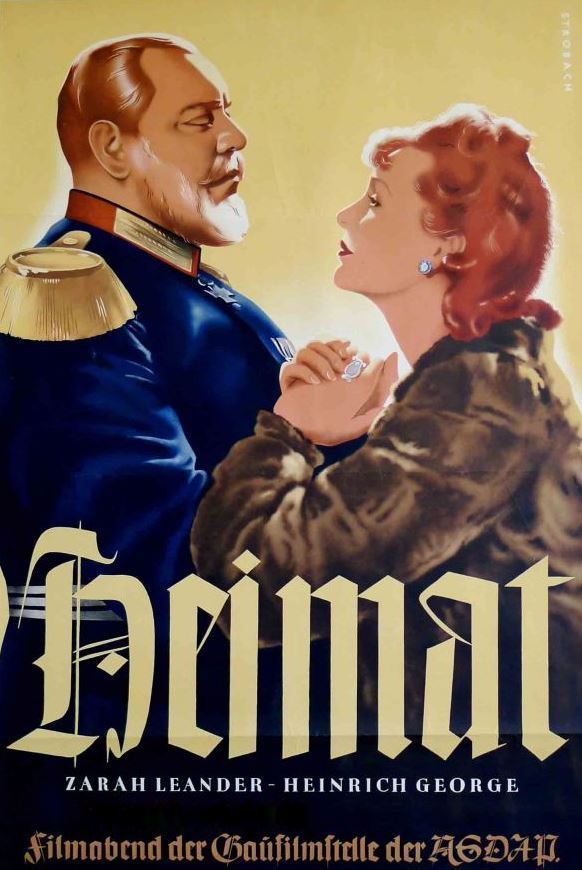The image is a vintage-styled, color-illustrated book cover with a portrait orientation. Dominating the top half of the cover is a detailed illustration set against a gold background. On the left side, there's a man with red hair and a white beard, dressed in a blue military uniform featuring gold epaulets and a red stand-up collar. He is gazing down at a woman on the right. The woman, with red hair elegantly pulled atop her head, wears a brown fur jacket and round diamond earrings. Her hands are interlocked, and she gazes up at the man. Across the bottom half of the illustration, the title "Heimat" is written in gothic script in gold. Below that, in white text, are the names "Zara Leander - Heinrich George." The bottom of the image contains another line of text in a foreign language.